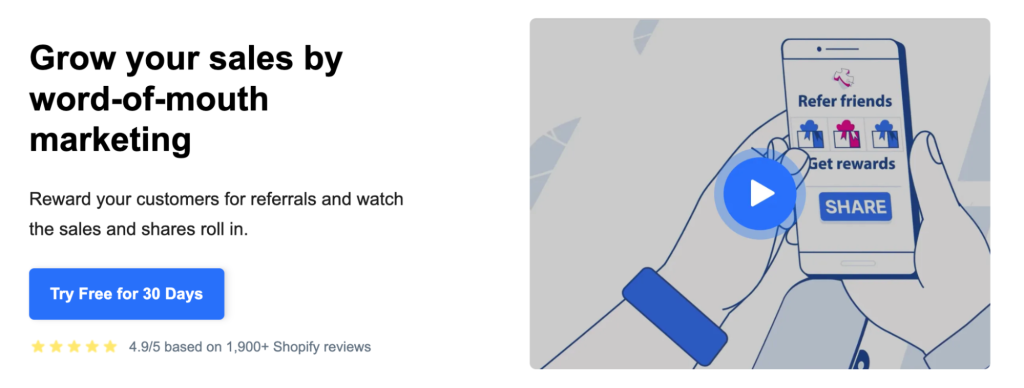This image is a clean, detailed screenshot of a mobile app advertisement. The ad features an animated video on the right side showing a person holding a smartphone. The screen of the smartphone displays the text "Refer friends, get rewards" along with a share button. The video is currently static, indicated by a play button overlaying it.

On the left side of the screenshot, bold black text reads, "Grow your sales by word-of-mouth marketing." Below this, in a smaller font, it says, "Reward your customers for referrals and watch the sales and shares roll in." Just beneath this text, there's a prominent blue button with white text that states, "Try free for 30 days."

Additionally, the ad showcases five yellow stars followed by the text "4.9 out of 5 based on 19,000+ Shopify reviews," highlighting the product's high customer satisfaction rating. The entire advertisement is set against a plain white background, creating a clean and unfussy visual presentation.